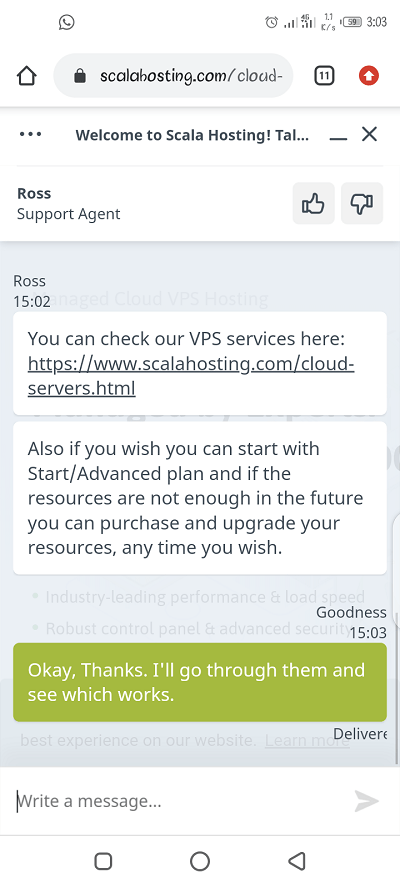Screenshot of a mobile webpage from Scala Hosting's website, specifically highlighting a live chat interface. At the top, the partially visible address bar reads "ScalaHosting.com/cloud...". Below the address bar is a dismissible notification banner with minimize and close options. Centered text in the banner reads "Welcome to Scala Hosting."

The live chat section features support agent "Ross" with the text "Ross, Support Agent" and thumbs up and thumbs down icons for feedback. The chat history shows Ross sending a message at 15:02, containing two text bubbles in white: 

1. "You can check our VPS services here" with an embedded link.
2. "Also, if you wish, you can start with the Start Advanced plan, and if the resources are not enough in the future, you can purchase and upgrade your resources anytime you wish."

User "Goodness" replies at 15:03 with a green chat bubble saying, "Okay, thanks. I'll go through them and see which works." At the bottom, the text input box is visible for further messages. The background of the chat interface is a light gray, providing a neutral backdrop for the conversation.